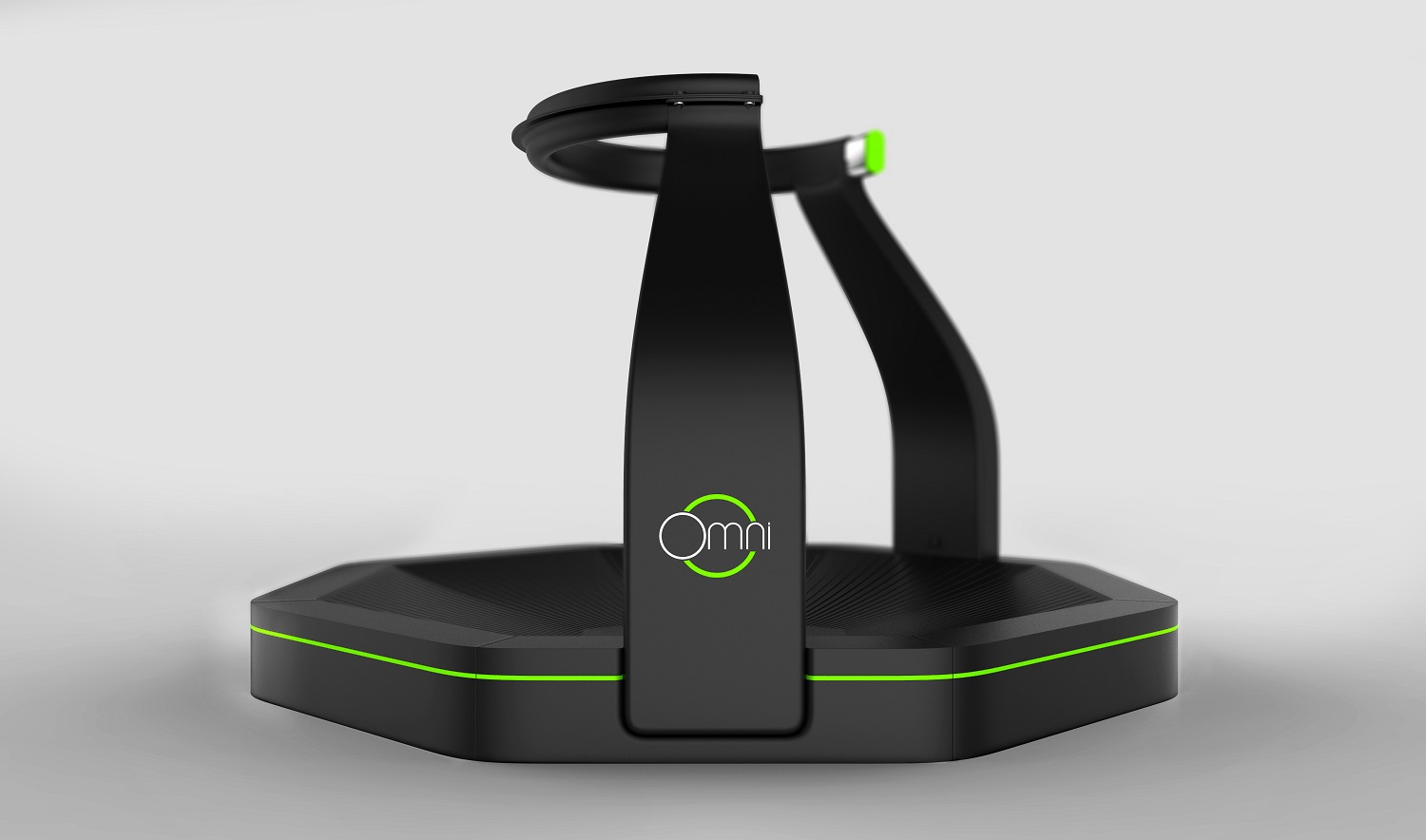This photograph showcases a VR (virtual reality) device known as an Omni Directional Treadmill. The device features a black hexagonal base adorned with a bright green stripe around its lower perimeter. Rising from two sides of the base are support arms that hold a ring typically positioned at the waist level of a user, enabling immersive movement within virtual environments. The base appears dark and shiny, while the background is a lighter gray, creating a contrast between the upper and lower parts of the image. Prominently displayed on one of the support arms is a logo—a green circle encircling the word "Omni" in white letters. Additionally, the device's edges and tips emit a bright neon green glow, enhancing its modern and futuristic appearance.